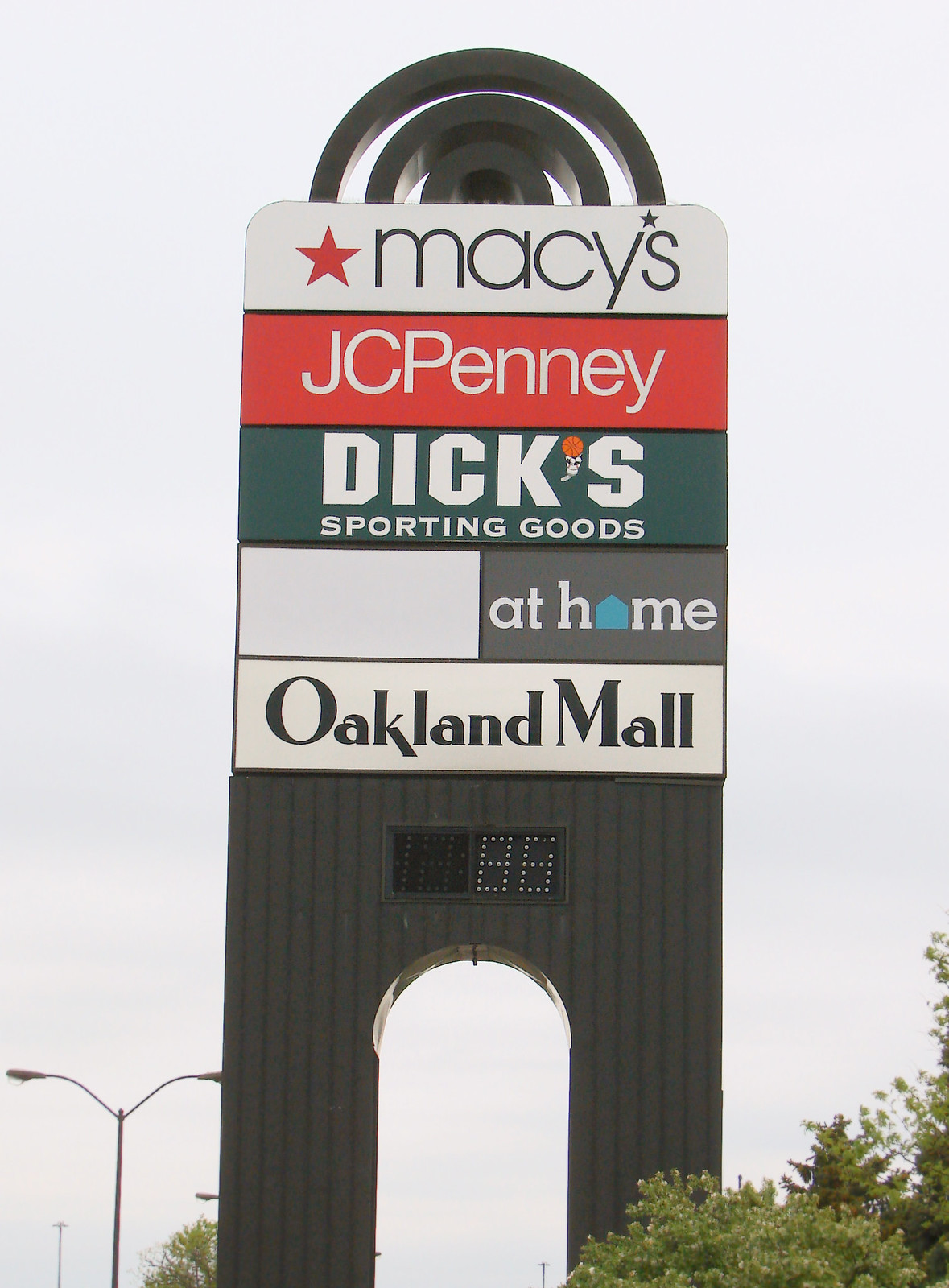This horizontal image captures the entrance sign to Oakland Mall from a low-angle perspective, emphasizing the sign's prominence against the sky. Located centrally from the bottom to the top of the photo, the sign stands tall in vertical orientation. Complementing the composition, there are double parking lot lights visible in the lower-left corner and a tree or shrub in the lower-right corner of the image.

The Oakland Mall sign is structured with distinct rectangular boxes that display store names. At the topmost position is Macy's, featured in black letters on a white background with a red star. Below Macy's, there is a red rectangle showcasing JCPenney in white letters. Next, in a full white rectangle, Dick's Sporting Goods is clearly stated in white text on a green background. Beneath these stores and central to the sign is 'Oakland Mall' written in bold black letters within a white rectangle.

An arch forms the lower center portion of the sign, directly above which an electronic board displays the temperature. Crowning the sign are three concentric black semicircles. The contrasting black and white design elements of the sign, apart from the red of JCPenney and the red star of Macy's, make each store name stand out vividly.